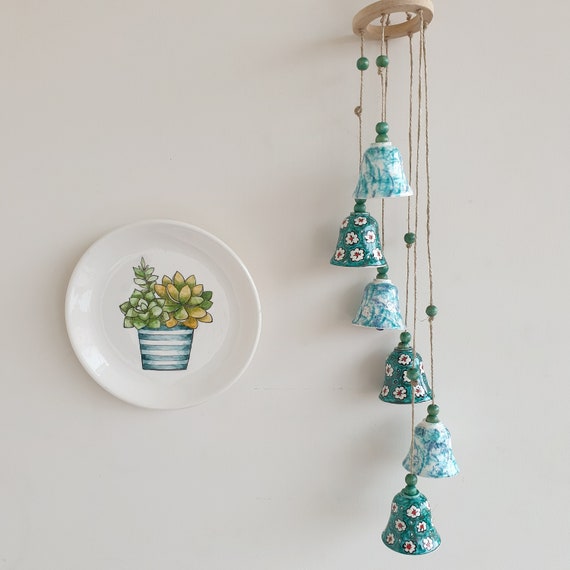The photograph captures a section of a gray wall with a white, decorative ceramic plate on the left side. The shiny, white plate features a blue and white horizontally striped pot in the center, holding three different types of succulents. The lush, green plants have hints of yellow in their leaves. To the right of the plate, there's a delicate wind chime hanging down, occupying nearly the entire height of the image. This wind chime has a light tan wooden ring at the top, from which six pieces of twine dangle in a spiral arrangement, descending from short to long. Strung on the twine are teal beads, and each end is adorned with ceramic bells. The bells alternate between two designs: one with a light teal brushwork, and the other a darker teal with white daisies and red centers, creating a charming and whimsical effect.